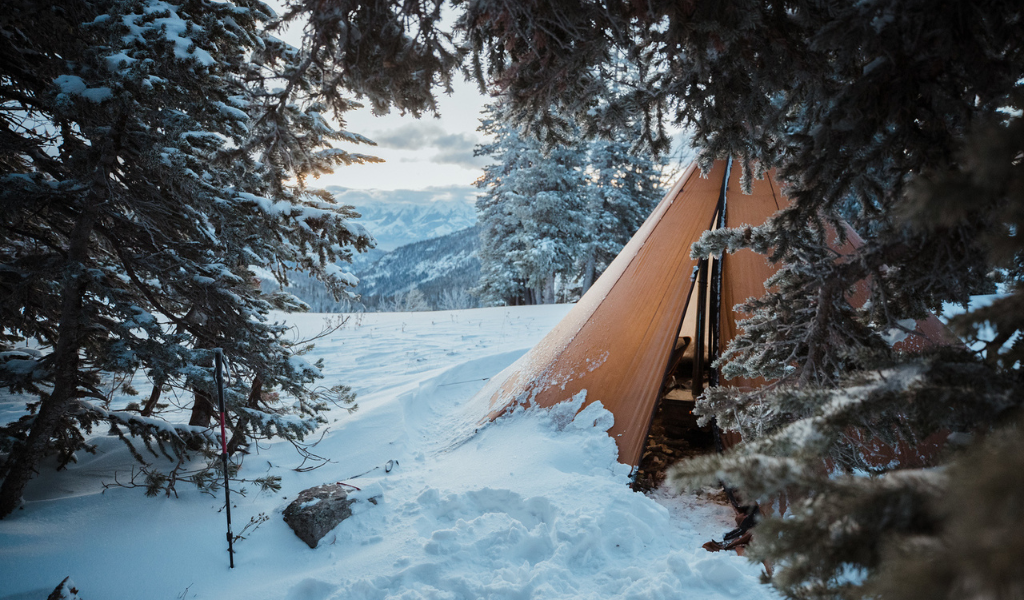The photograph captures a serene winter mountain scene bathed in daylight. The ground is blanketed in thick snow, and a light orange, triangular-shaped tent, reminiscent of a teepee, is prominently positioned in the foreground to the right. This tent has partially drifted snow along its side due to the wind and features a partially open door, revealing a well-lit, cozy interior with what looks like pillows and camping gear. Surrounding the tent are evergreen trees, heavily laden with snow, exhibited a dark brown hue that contrasts the white snow. Beyond the trees, distant mountains frame a tranquil valley, contributing to the expansive and picturesque backdrop. The presence of faint tracks in the snow adds a touch of human element to this otherwise undisturbed winter wonderland.